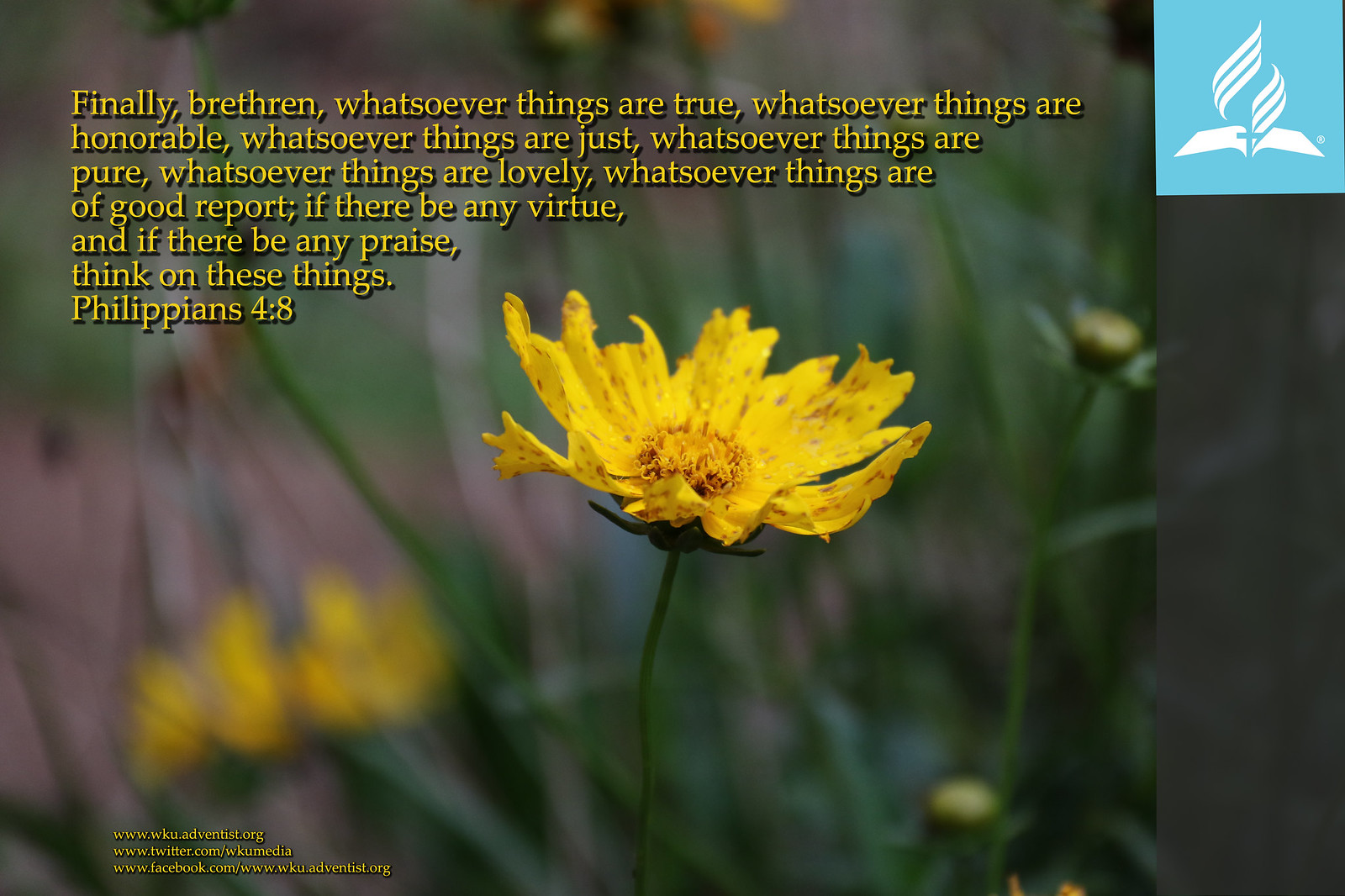This high-resolution photograph features a yellow flower, likely a daisy, with petals that appear slightly weathered, possibly from rain or hail. Dark spots speckle the petals, adding character to its natural beauty. The background is blurred, showcasing additional flowers and green grass, enhancing the focus on the primary bloom. 

In the top left corner, a yellow text overlay features an inspirational quote from Philippians 4:8: "Finally, brethren, whatsoever things are true, whatsoever things are honorable, whatsoever things are just, whatsoever things are pure, whatsoever things are lovely, whatsoever things are of good report, if there be any virtue and if there be any praise, think on these things." 

The upper right corner includes a blue logo depicting an open book with a cross. In the bottom left corner, there are small yellow hyperlinks, though they are too tiny to decipher. Overall, the image combines elegance and inspiration, emphasizing themes of beauty and virtue intertwined with nature.